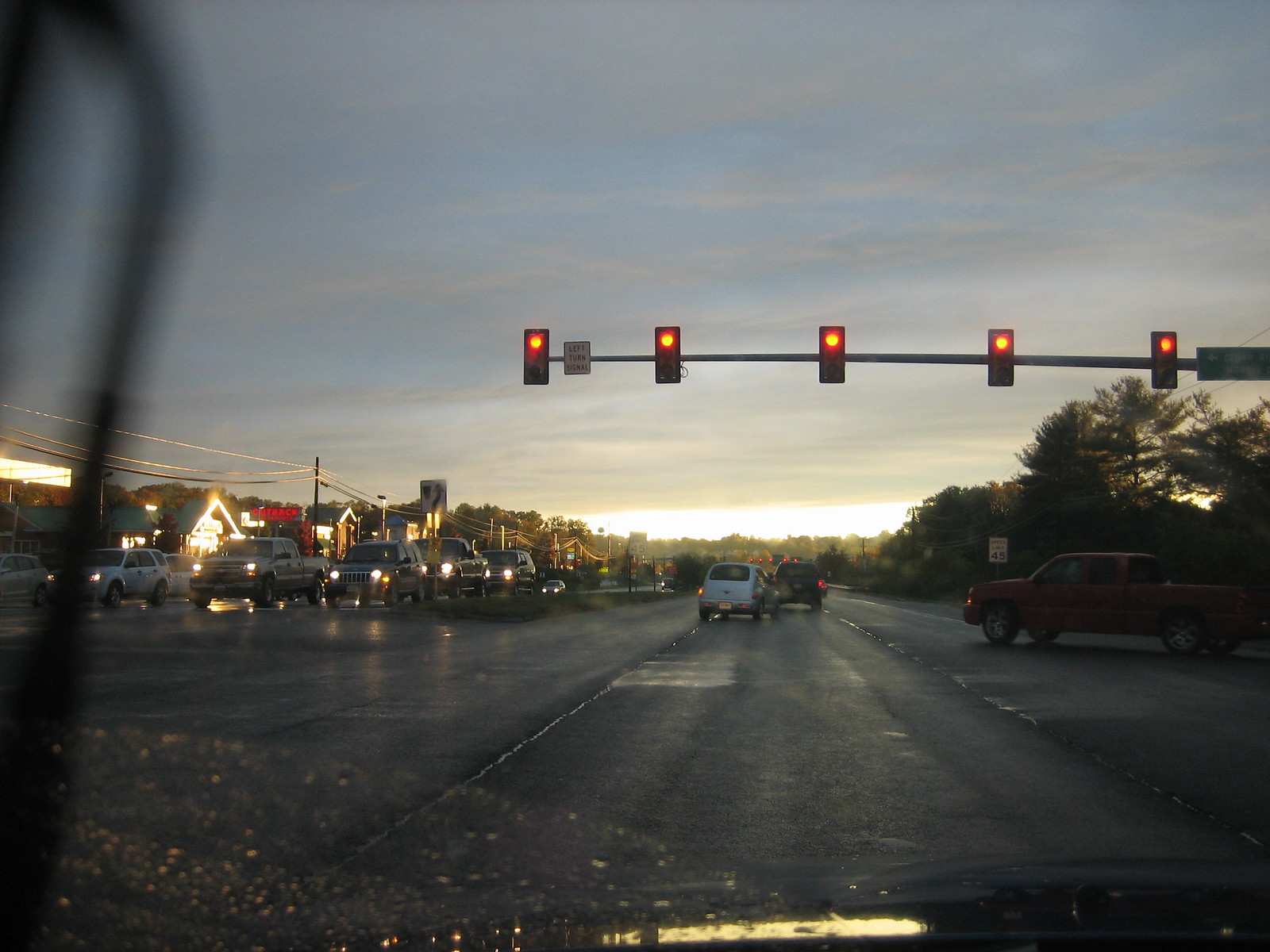The photograph offers a point-of-view perspective from within a vehicle stopped at a red traffic light, capturing a vivid urban scene through the front windshield. Dominating the center of the frame are five traffic lights, all glowing red, symbolizing a moment of stillness amid the bustling street. Directly ahead, two cars, one silver and the other dark-colored, are also waiting for the light to change. From the right side of the image, a red pickup truck is seen making a turn across the car's path. 

Across the street, a line of vehicles with their headlights on disperses light reflections on the damp pavement, hinting at recent rainfall. Water droplets cling to the windshield, with a clear pattern where the wiper has cleaned the surface, most notably on the bottom left. The street is flanked by a mix of houses and businesses, adding to the urban ambiance. This detailed snapshot encapsulates a moment of transit in a rain-kissed cityscape.